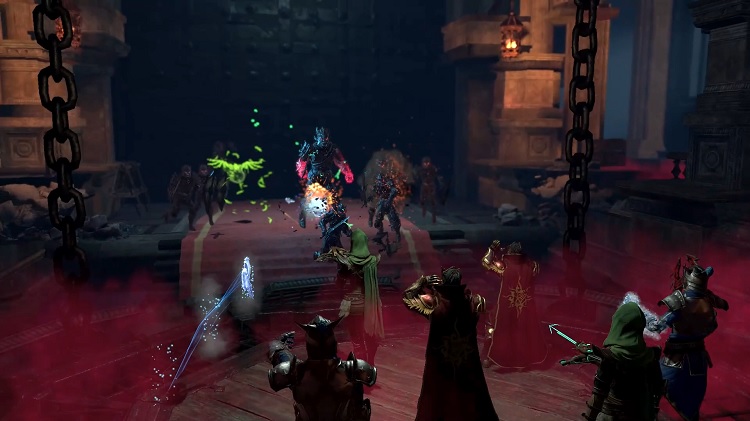This detailed scene, seemingly from a medieval-themed RPG video game, showcases a dramatic showdown in a dimly lit castle. The image captures six characters, their backs turned to us, standing on a wooden circular platform surrounded by an eerie red mist. Different characters are cloaked in diverse wardrobes—some in knight's armor, others with red capes, and a couple in green hoods, one of whom is wielding a bow and arrow. They're equipped with various weapons, possibly swords or crossbows, and appear to be casting spells.

Ahead, a set of carpeted stairs leads up to a different platform, where the opponents, including foot soldiers with shields, stand guard. Dominating this upper platform is a formidable figure in dark armor, with glowing pink or red hands, resembling a black knight. The setting is further accentuated by large chains hanging from the ceiling and dim lanterns illuminating the scene. The overall atmosphere is one of impending battle, with magical and physical confrontations about to unfold.